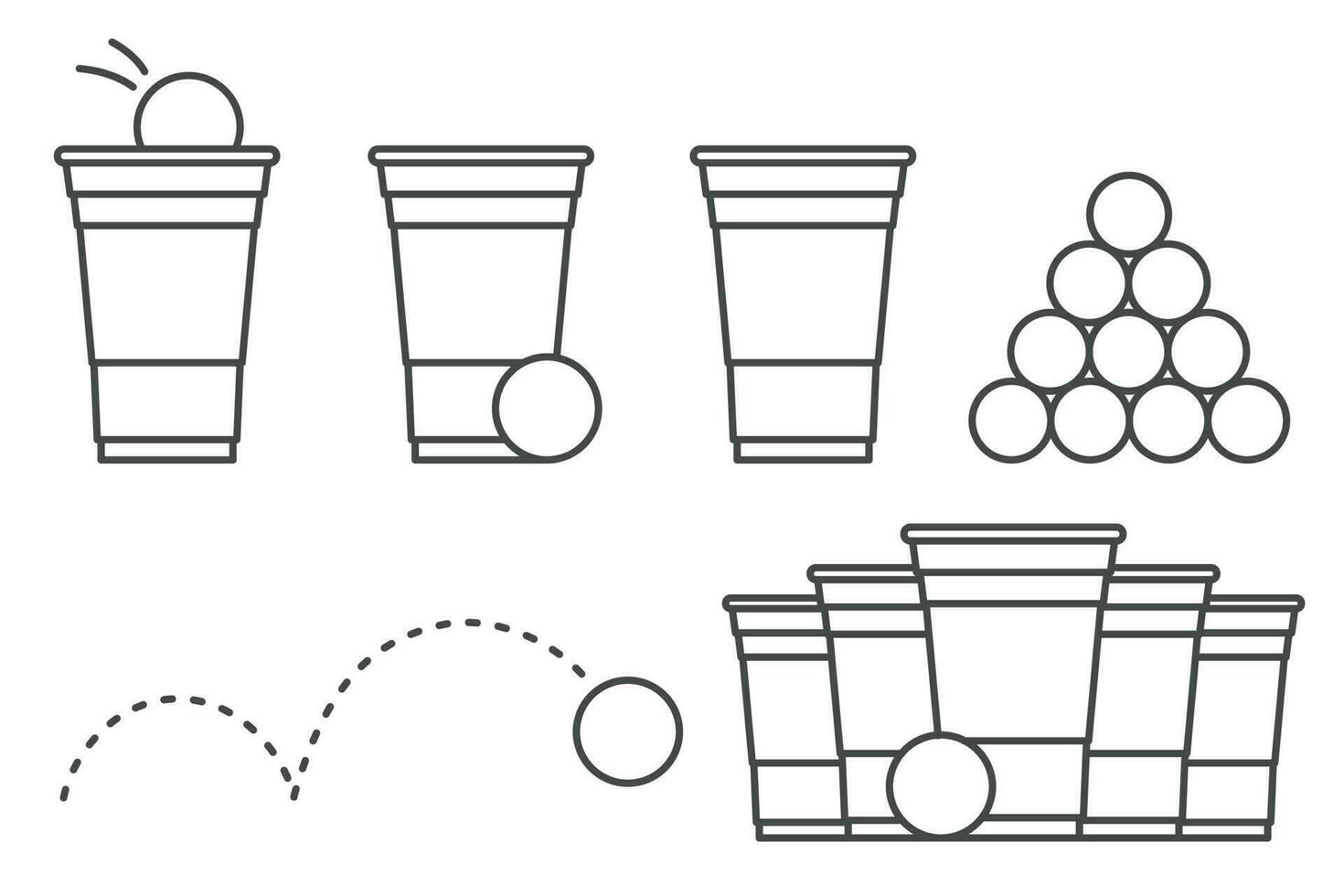This black and white illustration depicts a beer pong game setup. The top row features three colorless cups outlined in black. The first cup has a ping pong ball bouncing into it, while the second cup contains a ball at its base. The third cup is empty, and to its right is a neatly arranged pyramid of ping pong balls: one ball at the top, two below it, three in the third row, and four at the base. The bottom row showcases a series of graphics, including a dotted line showing a ball's bounce trajectory. Further to the right, there is a formation of five cups, with one cup in the front center, flanked by two cups set slightly behind on either side, giving the impression of an ascending arrangement. Additionally, a single ball rests at the bottom near the central front cup.